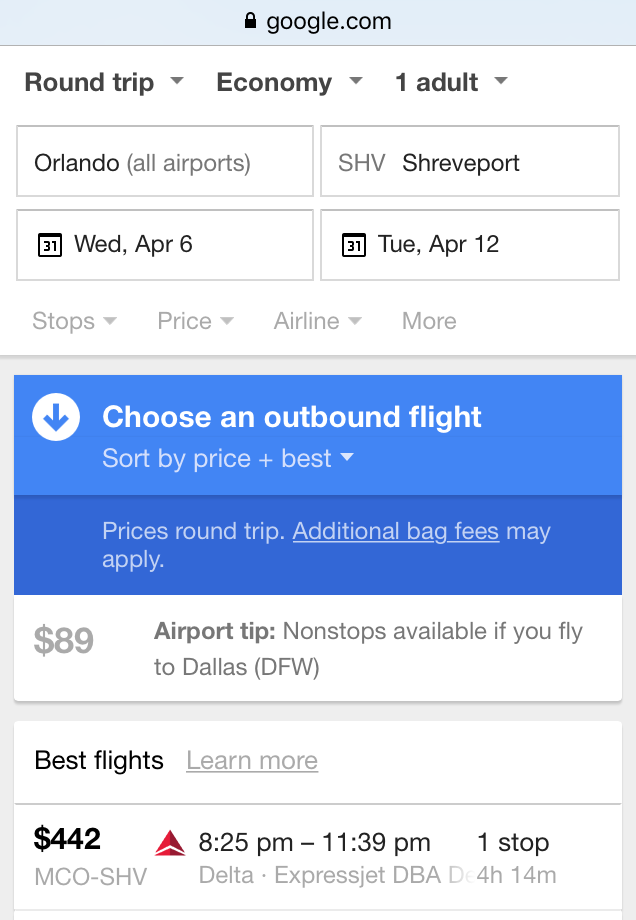This screenshot captures a flight booking interface, presumably accessed via Google Chrome, as indicated by the "google.com" browser tab at the top. The interface prominently features three tabs labeled "Round trip," "Economy," and "Adult," denoting the type of flight booking being searched. The user is looking for a flight from Orlando to Shreveport, with the departure date set for April 6th and the return flight on Tuesday, April 12th.

Further down the interface, there are filtering options labeled "Stops," "Price," "Airline," and "More," which allow users to refine their search criteria. A distinctive blue banner beneath these filters reads "Choose an outbound flight," with an option to sort results by "Price + Best." A note indicates that the prices listed are for round-trip tickets and that additional baggage fees may apply. The page highlights an airport tip amounting to $89 and lists the best flight option at a cost of $442.